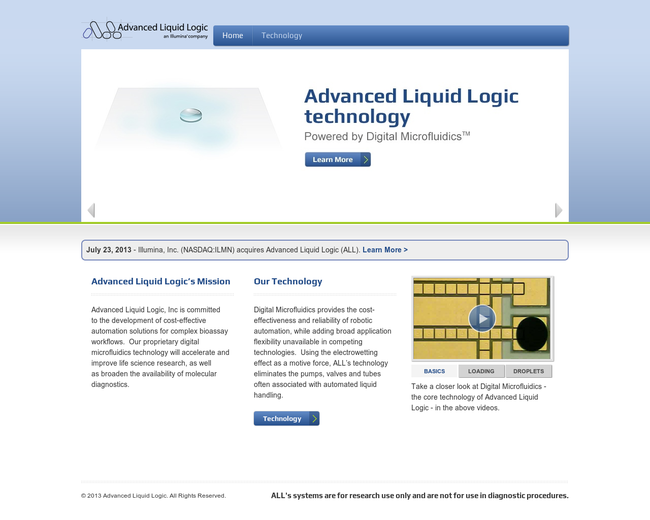The image shows a detailed screenshot of the homepage for the website "Advanced Liquid Logic Technology." At the top left corner of the site, there is the company name "Advanced Liquid Logic" prominently displayed, accompanied by two logos. The website primarily uses a blue and white color scheme and features an organized layout with various blocks of text and an embedded video at the bottom right corner, labeled "Basics." 

Across the top of the homepage are navigation tabs including "Home" and "Technology." There is a prominent image of a gel supplement, which appears to be stacked and bears a striking resemblance to a blown-up balloon doll. The site banner reads, "Advanced Liquid Logic Technology, powered by Digital Microfluidics." Below, there is a "Learn More" button.

On the left side of the homepage, there are two main sections titled "Advanced Liquid Logic’s Mission" and "Our Technology." These sections detail the company’s commitment to developing cost-effective automation solutions for complex bio-easy workflows, and explain that their proprietary Digital Microfluidics technology accelerates and improves life science research while broadening the availability of molecular diagnostics. The website elaborates on how Digital Microfluidics provides the cost-effectiveness and reliability of robotic automation, with broad application flexibility not found in competing technologies. This technology utilizes the electro-wetting effect to eliminate the need for pumps, valves, and tubes commonly associated with automated liquid handling systems. The embedded video on the bottom right gives an overview of these technologies.

Overall, the homepage is designed to educate visitors on Advanced Liquid Logic’s mission and the innovative technology they provide, which is aimed at scientists and those interested in cutting-edge automation in life sciences. The website carries a professional tone, offering insights into their research focuses and technological advantages.